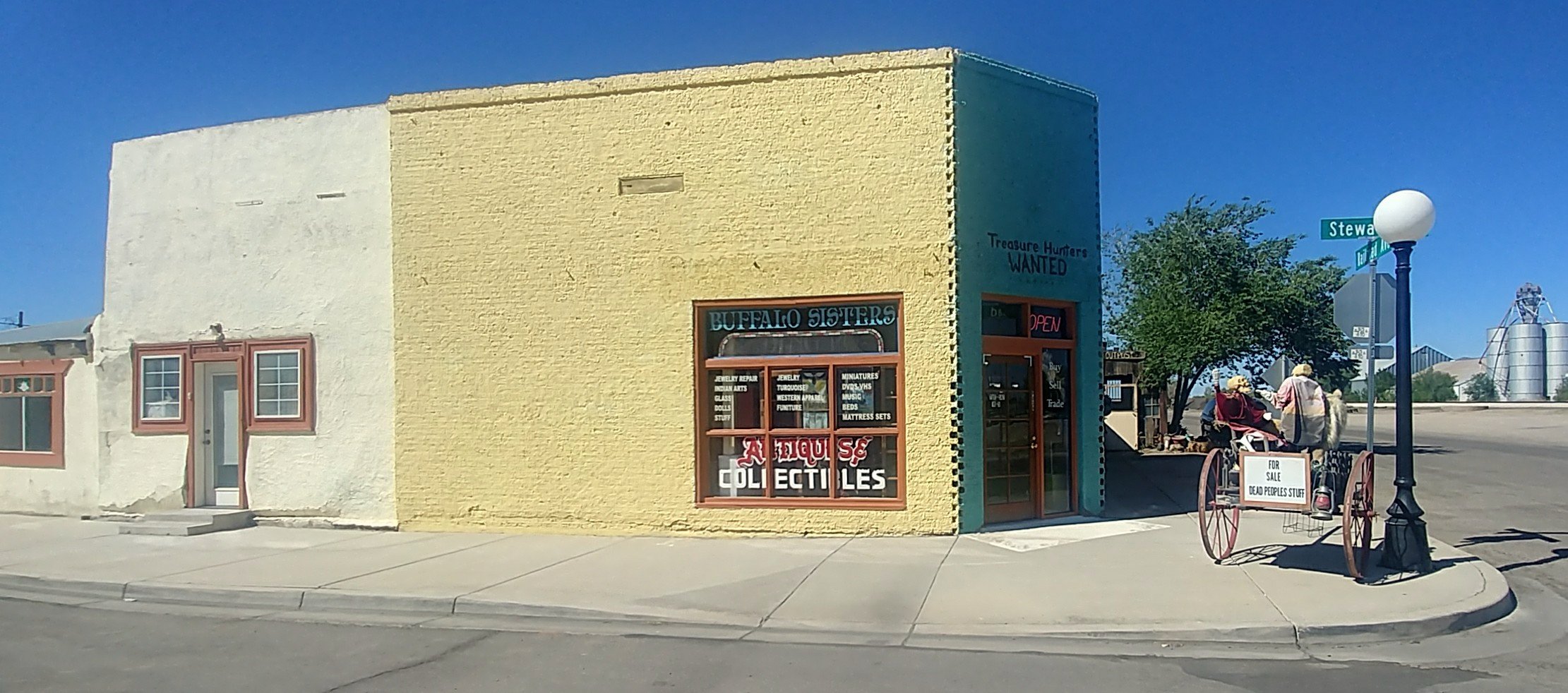This horizontally aligned rectangular photograph captures an old town scene, likely in middle USA, featuring a historic building situated on a street corner. The right section of the building is constructed of light brown bricks and adorned with several windows featuring distinctive red or dark brown trim. Prominently displayed on the top part of one window are the words "Buffalo Sisters" in white letters, while the bottom of the window bears the inscriptions "Antiques" in red and "Collectibles" in white. A lit "Open" sign is visible above the door, which is framed by additional small square windows and accompanied by a portion of the wall reading "Treasure Hunters Wanted."

The left portion of the building contrasts with its white stone façade, contributing to the vintage aesthetic. Pavement extends in front of the building, forming a large, light gray sidewalk alongside the street, which is constructed of asphalt. On this sidewalk, near the building's entrance and further enriching the nostalgic ambiance, stands a tall black lamppost topped with a circular white light. Adjacent to the lamppost, a green street sign is visible, partially reading "Stewart" in white letters.

Adding to the scene’s charm, an old-fashioned wagon with brown wheels sits in front of the entrance, displaying an unreadable white "for sale" sign. In the backdrop, a green-leafed tree and silver grain silos emphasize the rural setting. This photograph encapsulates the idyllic allure of a small-town antique shop, filled with relics and memories, inviting passersby to explore its treasures.